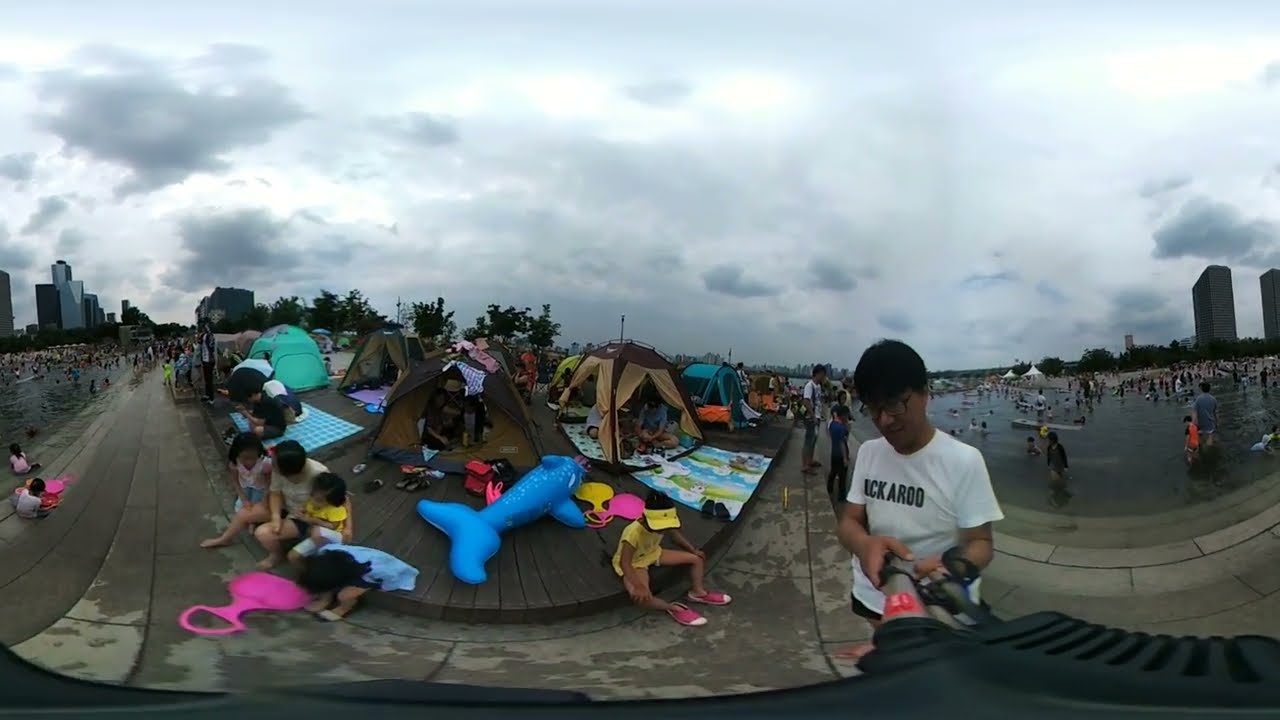The photograph captures a bustling outdoor scene with numerous details. The setting appears to be a man-made beach or waterfront area, characterized by a central walkway lined with colorful tents indicating a camping area. This area is surrounded by water on both the left and right sides, with people wading and playing in the shallow waters, their bare feet splashing around. The water is framed by concrete steps giving it a structured, user-friendly look, transitioning to more natural beach-like edges further out.

The sky is heavily overcast with thick gray clouds, suggesting impending rain. In the background, the cityscape comprises large buildings—gray, white, and black structures—adding an urban feel to the scene. Trees and bushes with rich green foliage are visible, contributing to the natural elements amidst the urban layout.

Among the crowd, a notable pair includes a young girl in a yellow t-shirt and visor, accompanied by a man in a white t-shirt, seemingly steadying a motorcycle. The ground before the tents appears wet, hinting at recent rainfall or residual moisture from the waterfront. The vibrant array of tents includes blue, brown, beige, and greenish hues. There are also playful elements like blue floaties shaped like dolphins.

In summary, the photograph presents a vivid juxtaposition of urban and natural elements in a highly active waterfront area filled with people camping, playing, and enjoying the outdoors under a gray, cloud-filled sky.